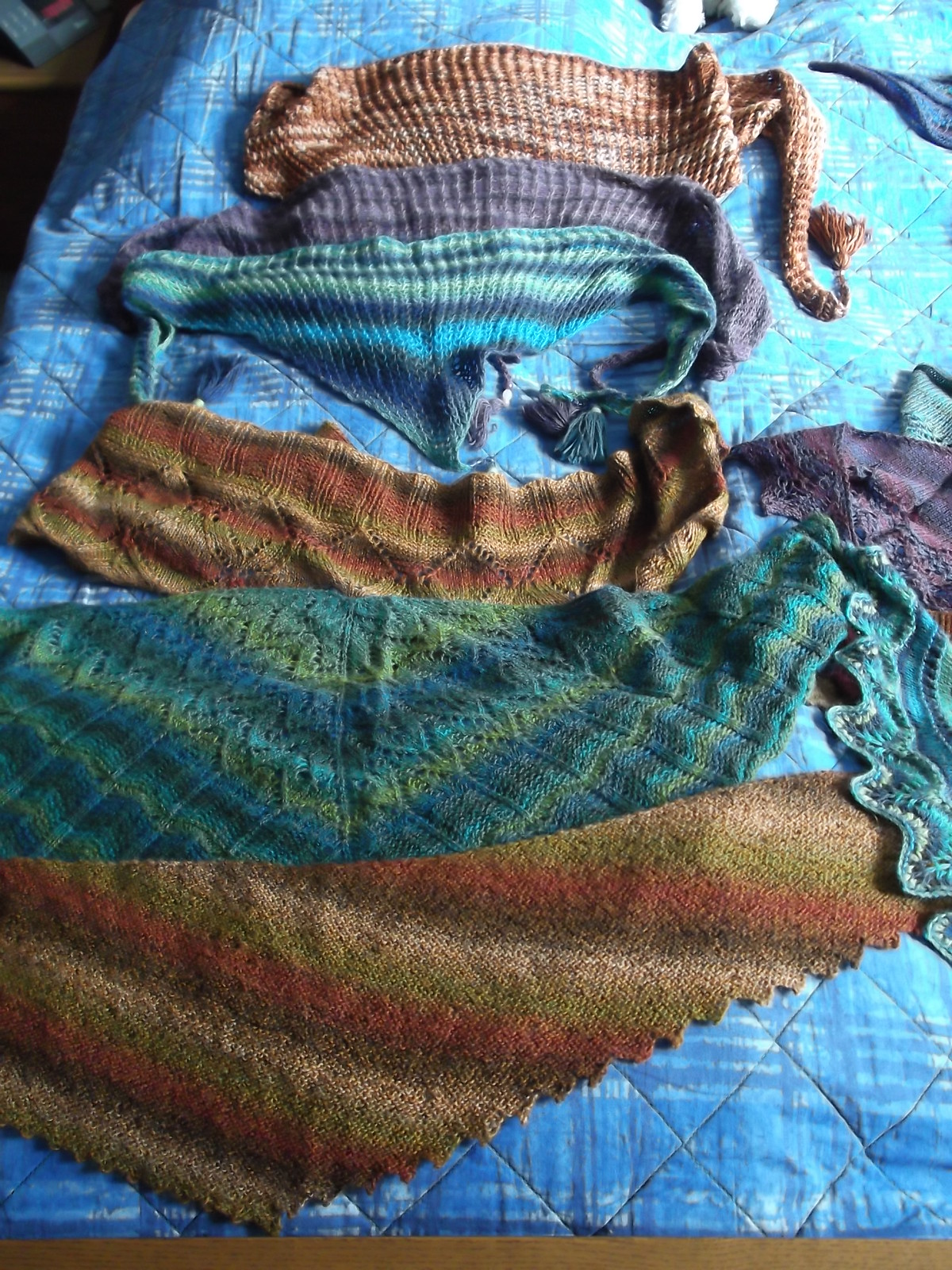The photograph captures an indoor scene featuring multiple pieces of crocheted fabric spread out over a predominantly blue bedspread adorned with white lines and darker blue stripes. The fabric pieces are arranged in a fan-like pattern, each roughly triangular and reminiscent of bandanas or scarves, with variously scalloped or straight edges. A notable detail in the upper part of the image is the presence of two tiny white paws, suggesting the possible presence of a live animal or a stuffed toy on the bed. Each fabric piece boasts unique multicolored patterns, showcasing a diverse palette: the bottom one features brown, olive green, beige, and red; the next is teal, aquamarine, and lime green; followed by one with red, olive green, beige, and brown; then comes a piece with dark blue, light blue, and light green tones. The subsequent scarf displays various shades of purple, while the one above incorporates tones of brown. Out of view to the right, additional fabric pieces are scattered. Moreover, the upper right corner of the image subtly reveals a side table with a picture frame, adding a touch of homeliness to the scene dominated by the creative, colorful textiles.